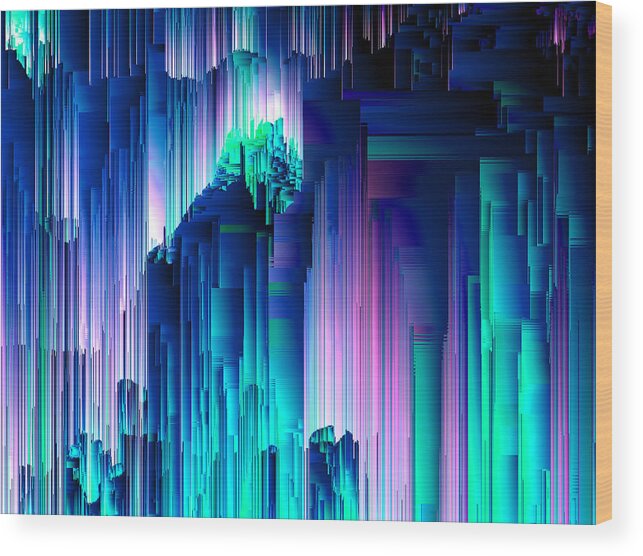This is a highly detailed, computer-generated image that non-representationally portrays a complex pattern of overlapping vertical strokes. These strokes, all parallel but varying in width and color, form an intricate tapestry that somewhat suggests architectural forms, like a castle up on a cliff. The vertical strokes are striated with slightly curved horizontal lines, evoking the impression of cylindrical pillars. The colors used range from neon pink to various shades of teal, aqua, blue, and violet. The image is a large, wide, vertical rectangle set against a white background and bordered on the right side by a woodgrain-like strip, giving it a three-dimensional appearance as though the painting is angled slightly to the left, revealing the light brown edge of the board it is "painted" on. Overall, the artwork is a mesmerizing blend of purples and blues with varied interruptions and continuations in the lines, enhancing its depth and complexity.